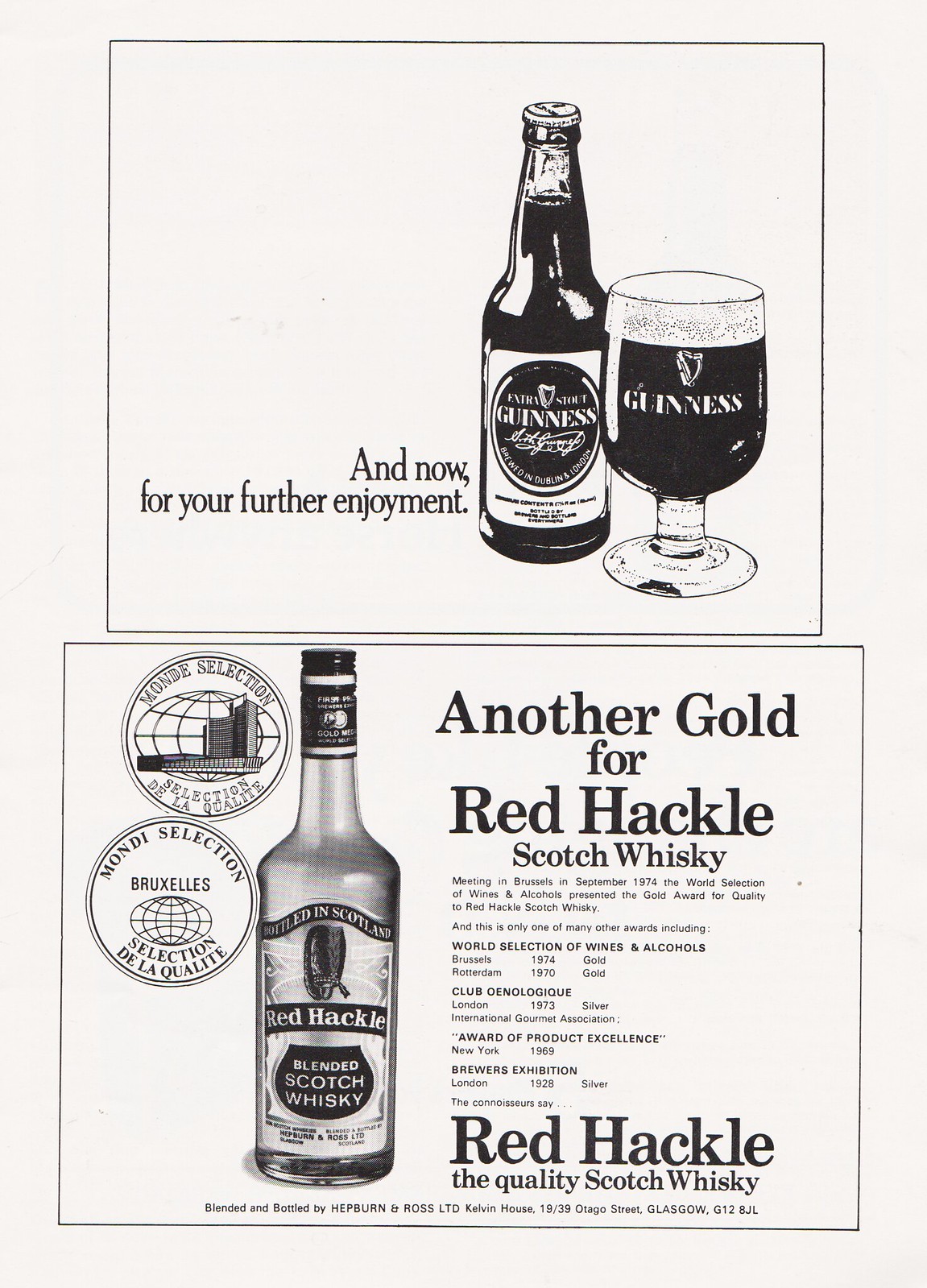This image, reminiscent of a vintage magazine advertisement page, is framed with a thin black border on an off-white, slightly textured background. The rectangular ad is divided into two separate sections by a black line. The top section features a detailed illustration of a bottle of Guinness beer still capped, accompanied by a frothy, full pint glass etched with the word "Guinness." Beside the illustration, a caption reads, "And now for your further enjoyment."

The bottom section advertises Red Hackle Blended Scotch Whiskey, prominently displaying a black-and-white photograph of the bottle. Above the bottle, in bold text, is the headline, "Another Gold for Red Hackle Scotch Whiskey," referring to the Gold Award for Quality received at the World Selection of Wines and Alcohols held in Brussels, September 1974. Additional accolades for Red Hackle are listed, including awards from Rotterdam 1970, London 1973, and New York 1969, highlighting the whiskey's celebrated quality. Furthermore, it mentions the distillers, Hepburn and Ross, Ltd., with the address Kelvin House, 19/39 Otago Street, Glasgow G12 8JL.